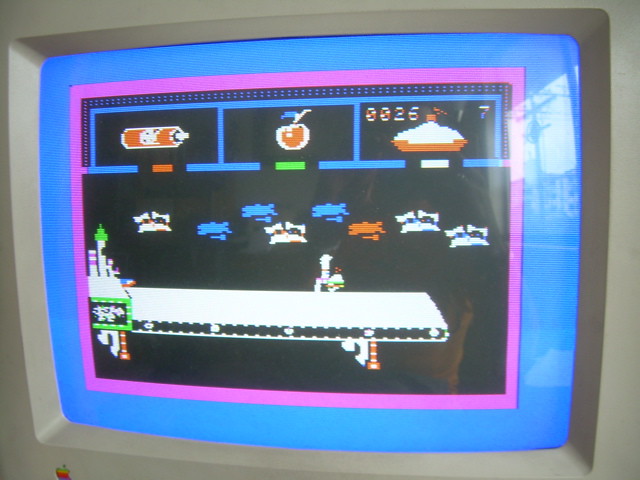The image features a vintage, white computer monitor typical of the early 1980s design. The left-hand side of the monitor displays the iconic Apple logo in its classic rainbow color scheme, featuring visible segments of green, white, orange, and red hues. The screen showcases an old-school video game characterized by a layered border design: an outer blue border followed by a purple border framing the gameplay area. The game itself has a black background and portrays what appears to be a retro, 1980s-style space or naval battle. The game elements include blue, orange, and white ships, along with a white line strip. In the upper right-hand corner, there is an orange and white object resembling a pie chart or indicator.